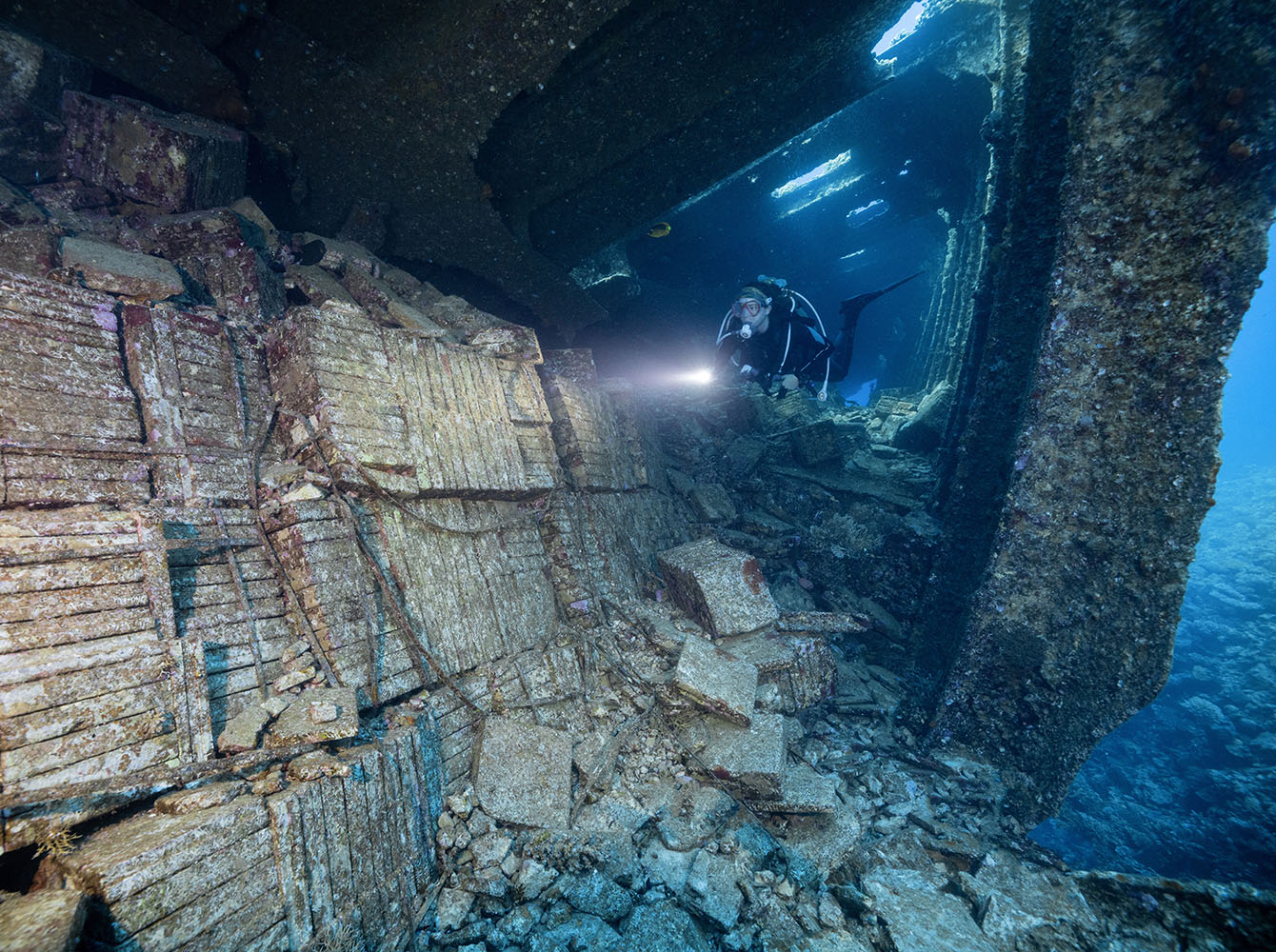A scuba diver explores an underwater shipwreck, equipped with black swimming fins and red-outline goggles. The diver, holding a flashlight, has a mouthpiece connected to an oxygen tank. Surrounding the wreck are numerous rocks and bricks, characteristic of the ship's remains. The wreckage appears dark brown and black, overgrown with algae and rust, with green and white patches indicating advanced deterioration. The water in the lower right-hand corner reveals other living organisms and rocks scattered across the seabed, adding to the scene's enigmatic underwater biodiversity.